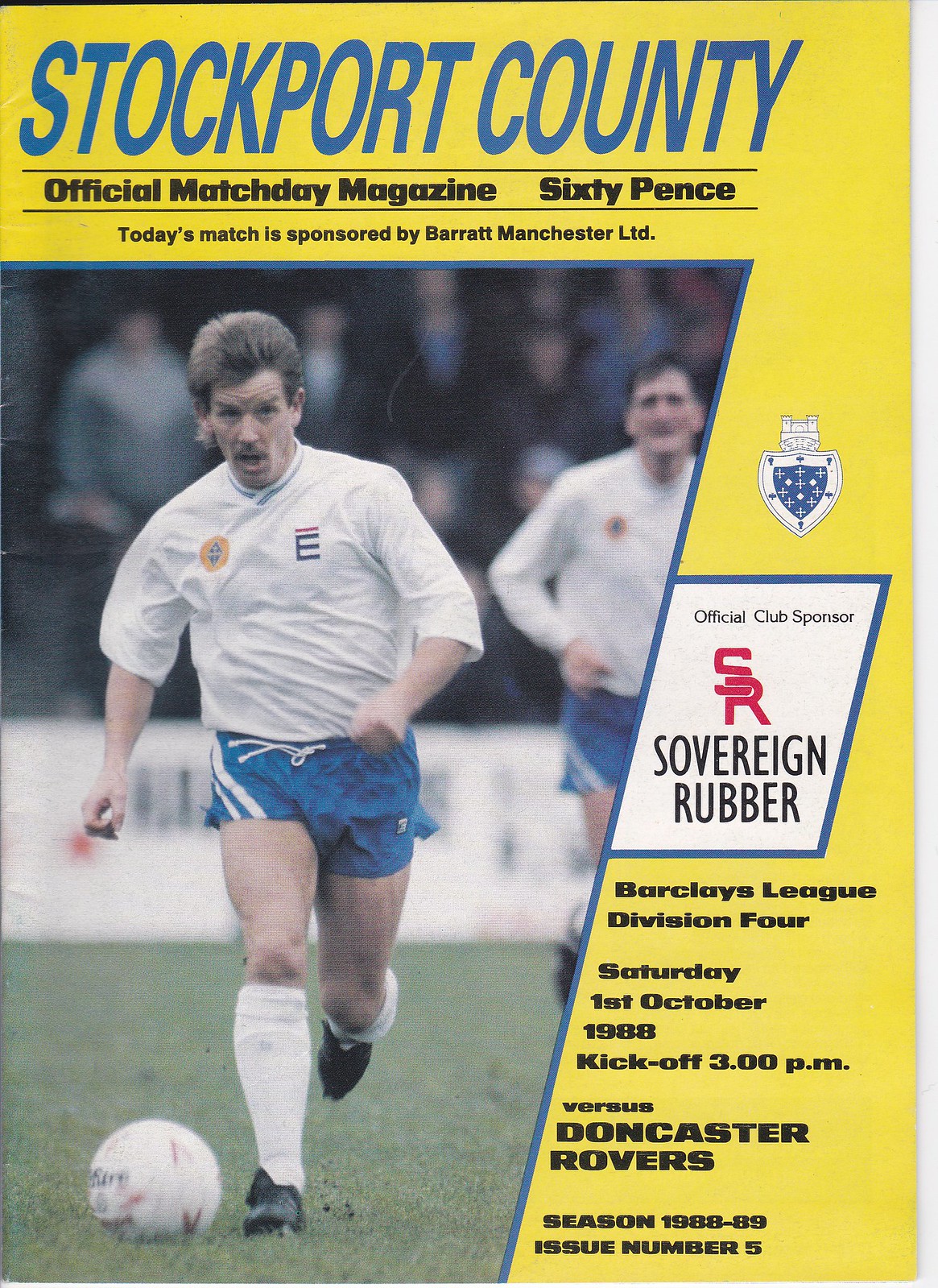The image is a rectangular cover of an old magazine titled "Stockport County Official Match Day Magazine," priced at 60 pence. It predominantly features a photograph of a white male soccer player in an action pose, running with a white soccer ball in front of him. The player is dressed in a white short-sleeved shirt, blue shorts, and white knee-high socks. Another player in the same uniform is blurred in the background, and there appears to be an overcast sky suggesting diffused sunlight.

The magazine has a yellow background at the top and right-hand sides. At the top, "Stockport County" is written in blue print. Below it, a thin horizontal line separates it from the text "Official Match Day Magazine, 60 pence" in black, followed by another black horizontal line. Beneath these lines, it reads, "Today's match is sponsored by Barrett Manchester LTD."

To the right of the photograph, within the yellow background, is a white shield with a blue outline. The shield features a castle on top and another blue shield with white crosses inside. Below this is a white parallelogram with a blue border, containing the text "Official Club Sponsor, Sovereign Rubber" in black, accompanied by the letters "S" and "R" linked together in red.

Further down, in black print, it states, "Barclays League Division IV, Saturday, 1st October 1988, kickoff 3:00 p.m. versus Doncaster Rovers, season 1988 to 89, issue number 5."